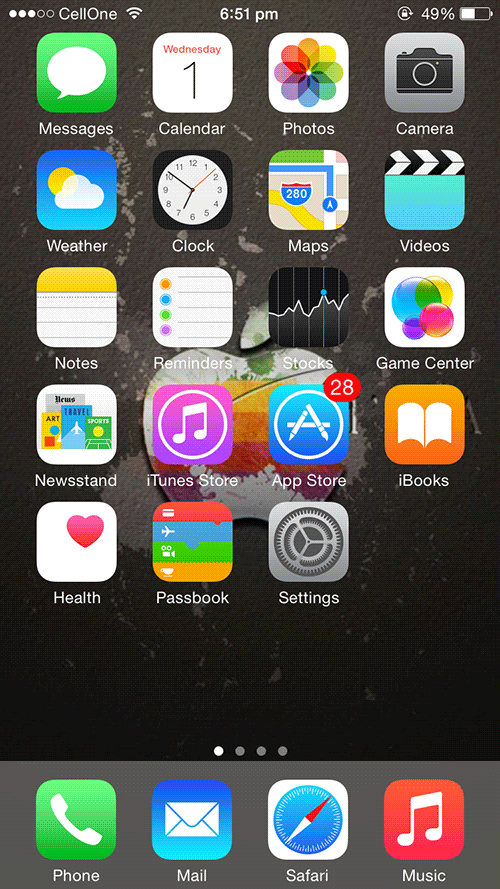Screenshot of an iPhone Home Screen:  

In the top left corner, the status bar displays the phrase "3 out of 5" alongside cell service indicators and a Wi-Fi signal. The current time is shown as 6:51 PM, and the battery icon on the right shows 49% remaining.  

The screen is filled with a 4x5 grid of app icons, neatly arranged in rows:  

- Top row: Messages, Calendar, Photos, Camera  
- Second row: Weather, Clock, Maps, Videos  
- Third row: Notes, Reminders, Stocks, Game Center  
- Fourth row: Newsstand, iTunes Store, App Store, iBooks  
- Bottom row: Health, Passbook, Settings  

Each app icon has the classic rectangular shape with rounded corners.

The background behind the apps features an abstract design with a central Apple logo accentuated by a paint splatter pattern, set against a black backdrop.  

Near the bottom center of the screen, there are four dots indicating multiple home screen pages, with the first dot highlighted, signifying the active page.  

At the very bottom, a dock contains four primary apps—Phone, Mail, Safari, and Music—each within its own gray background for easy identification.